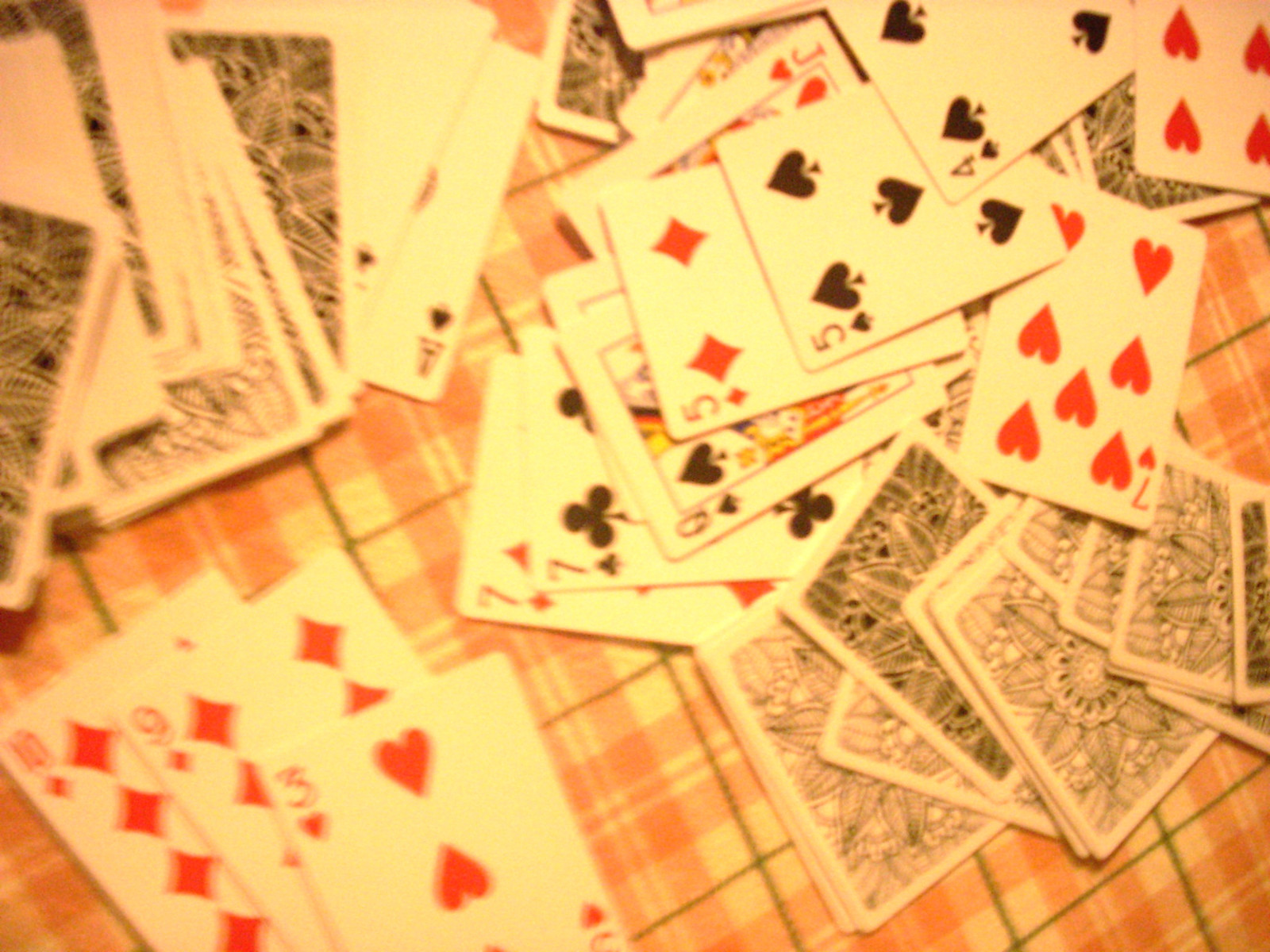This slightly out-of-focus photograph captures a chaotic array of playing cards scattered across a table adorned with a red and white checkered tablecloth. In the bottom left corner, three face-up cards are prominently visible: the ten of diamonds, nine of diamonds, and three of hearts—all in red. To their right, a stack of face-down cards displays backs adorned with a black sketch of a flower framed by a white border. Above these cards, several other face-up cards can be seen, including the seven of clubs, queen of clubs, five of diamonds, and five of hearts. Various other cards, some face-up and others face-down, are haphazardly arranged in multiple piles, adding to the disorganized appearance. The blurry quality of the image makes it challenging to identify some of the cards.